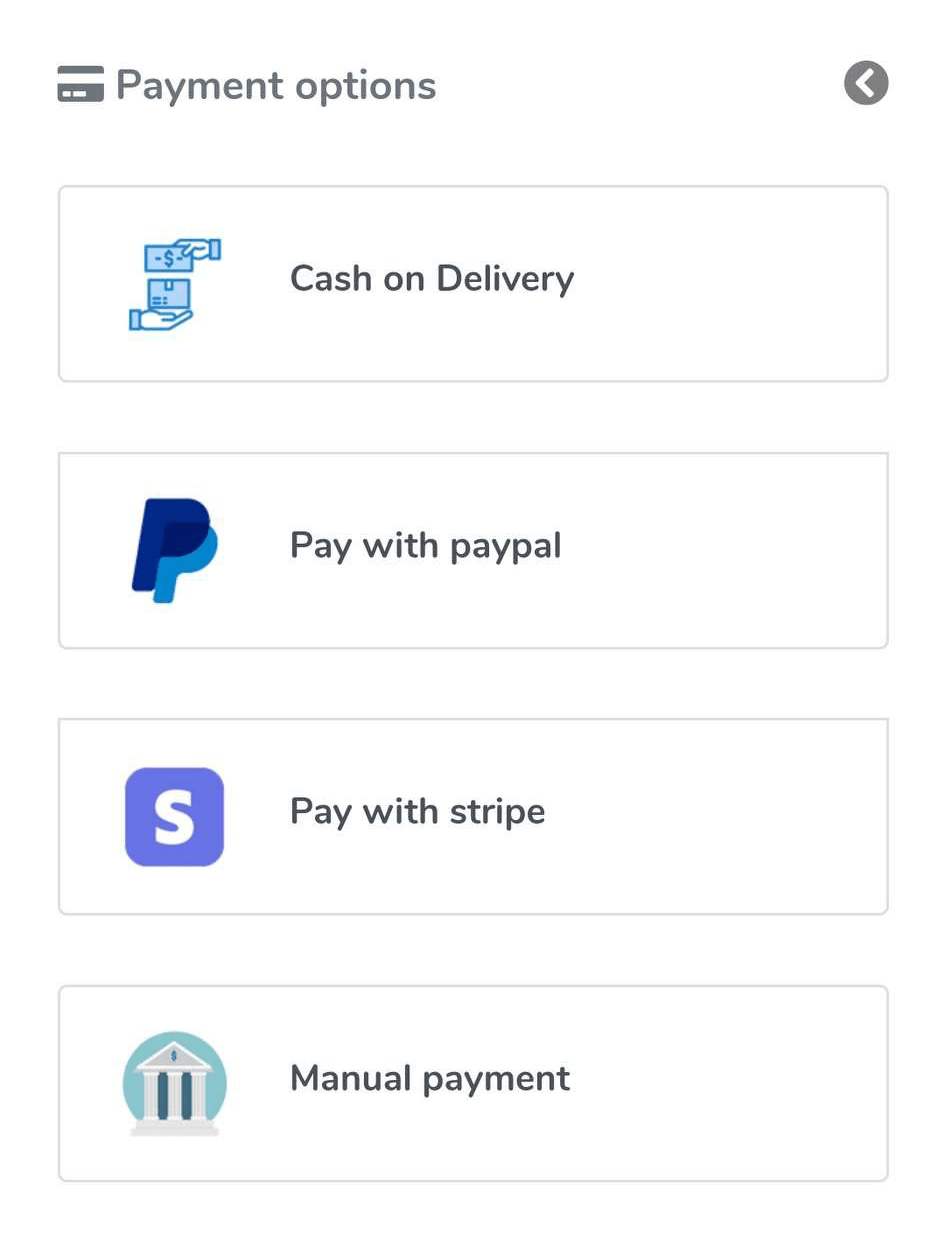This is a screenshot of a payment options page, featuring a clean and straightforward layout. At the top, there is the header "Payment Options," displayed in gray lettering with a small credit card icon situated to the left and a gray back button to the right. The menu has a white background and uses black lettering for enhanced readability.

Below the header, there are four distinct payment options:

1. **Cash on Delivery (COD)**: Illustrated by an icon depicting two hands, one handing over cash to the other, symbolizing an in-person transaction upon item delivery.

2. **Pay with PayPal**: Accompanied by the recognizably blue PayPal logo, offering a secure online payment option.

3. **Pay with Stripe**: Includes the Stripe logo, representing another secure online payment gateway.

4. **Manual Payment**: Represented by an icon of a classical building with large pillars and a cash symbol on top, reminiscent of a Roman-style bank, suggesting a traditional bank transfer method.

Overall, this page is designed to provide users with a clear and easy-to-navigate selection for completing their payments.